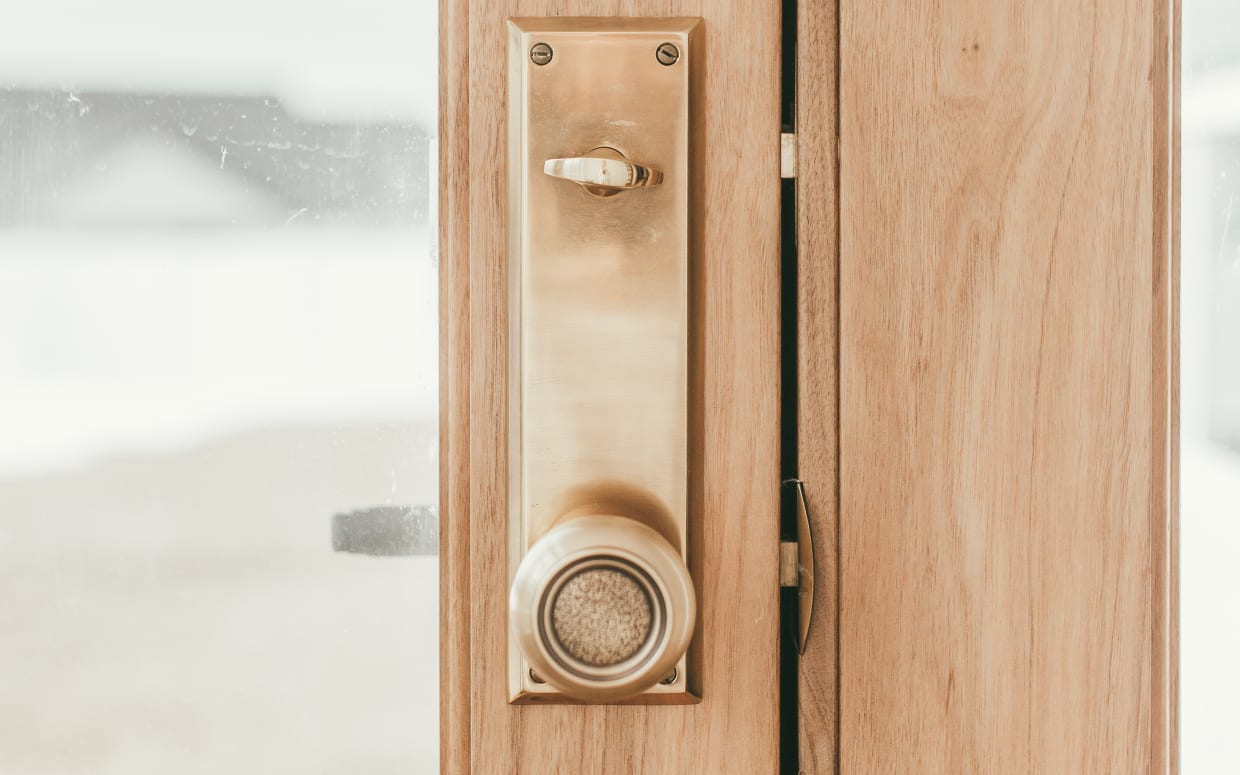This close-up image captures a door made of unfinished tan oak with a matching frame on the right. The door features a substantial brass lock plate, secured with four brass screws, and a multi-functional locking system. The top part of the plate hosts a security lock reminiscent of a bird beak, pointed at nine o'clock. Below, a large rectangular brass block integrates a classic round doorknob at the bottom. The door's internal mechanisms include a brushed aluminum finish on the inside and a shinier exterior aluminum casing. Through a pane of glass in the door, a lever-type outside knob is visible, contrasting with the regular round knob inside. The backdrop reveals soft, neutral colors suggesting an outdoor scene with parts of a house, possibly eaves, a street, and an ambiguous lawn or dirt area in the distance, creating a serene and understated atmosphere.